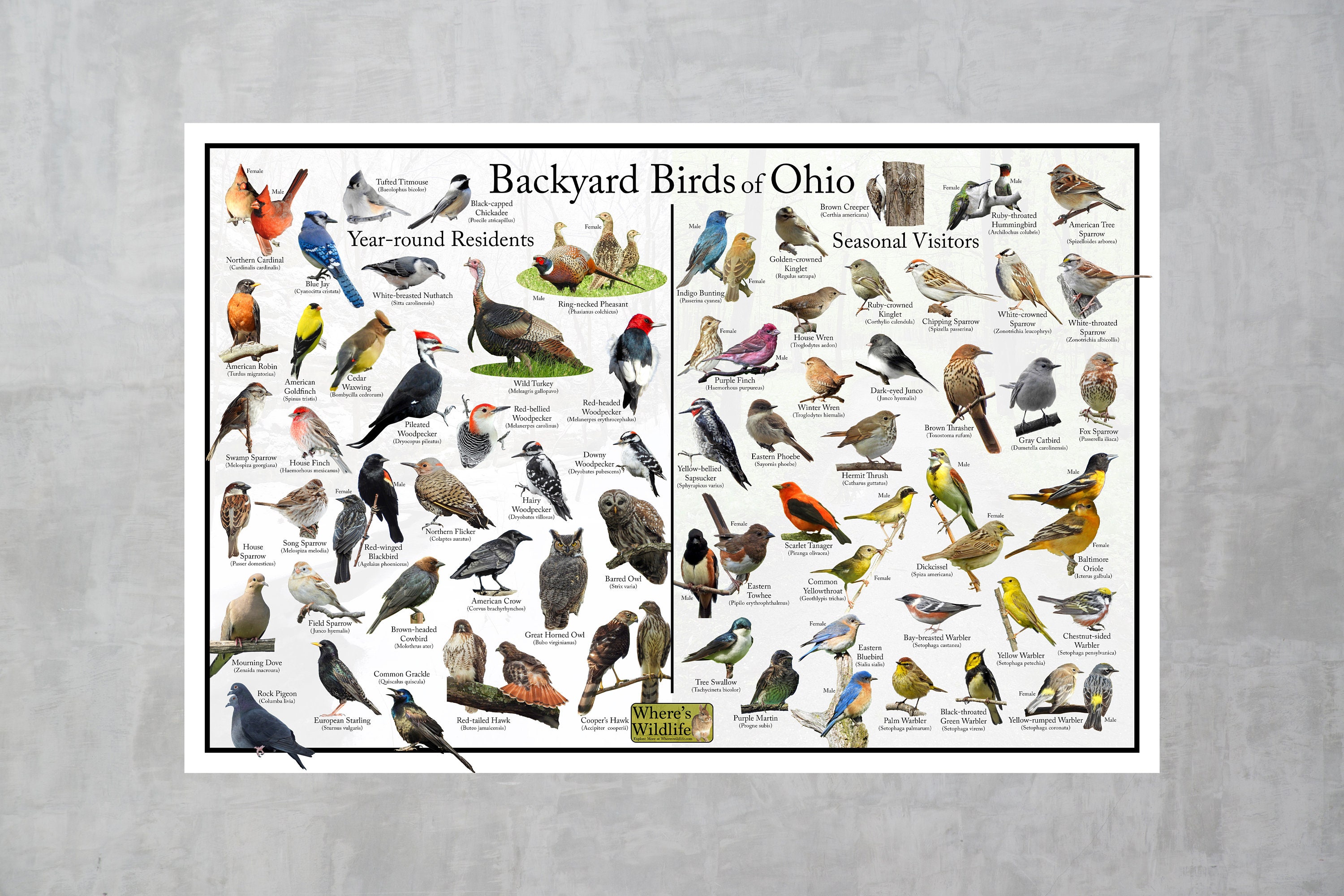The image showcases a detailed illustration titled "Backyard Birds of Ohio," featuring a large graphic with 30 to 40 vibrantly colored birds. The page is divided into two sections: the left side displays the year-round residents, while the right side highlights the seasonal visitors. The birds range from common backyard species such as blue jays, cardinals, robins, and woodpeckers to larger birds like turkeys and owls. Each bird is accompanied by its name, scientific name, and common nomenclature. The illustrations also incorporate natural elements; woodpeckers are shown with trees, and some birds, like turkeys, are depicted with patches of grass. The birds exhibit a spectrum of colors, including blue, yellow, red, brown, and even purplish hues. At the bottom of the image, a gold emblem reads "Where's Wildlife?"